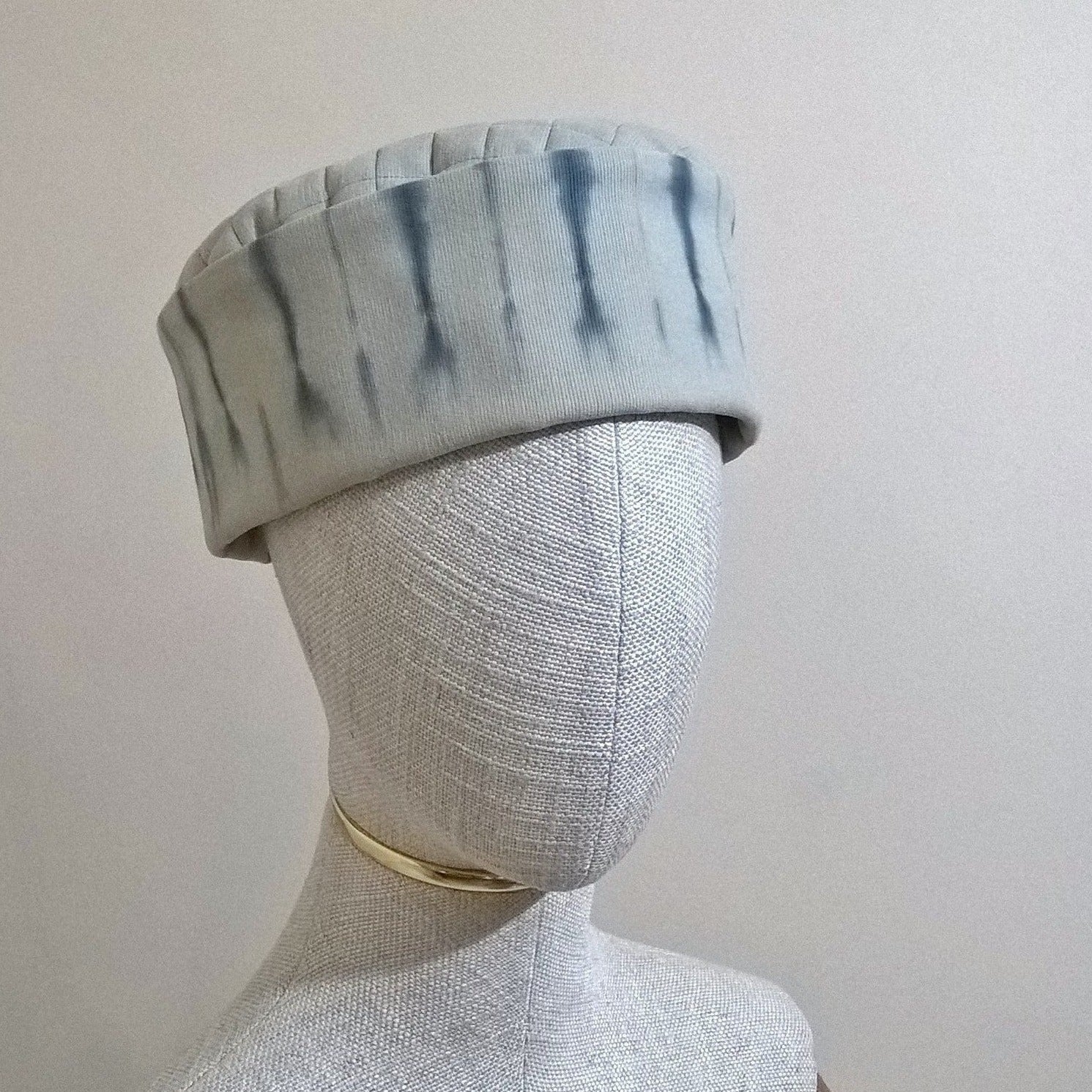This image features a fabric-covered mannequin bust cropped at the shoulders and posed against a grayish-white background. The mannequin is upholstered in gray fabric and has visible seams running up the middle of its face and chest and along the sides of its neck and shoulders. Adorning the mannequin’s neck is a tight-fitting gold choker necklace. Atop the mannequin’s head sits a unique, boutique-style hat resembling a quilted, Russian-style beanie. The hat is predominantly an off-white color with faded, denim-like navy blue tie-dye patterns and lighter quilting at the top. The mannequin has no facial features, emphasizing the accessories it displays.